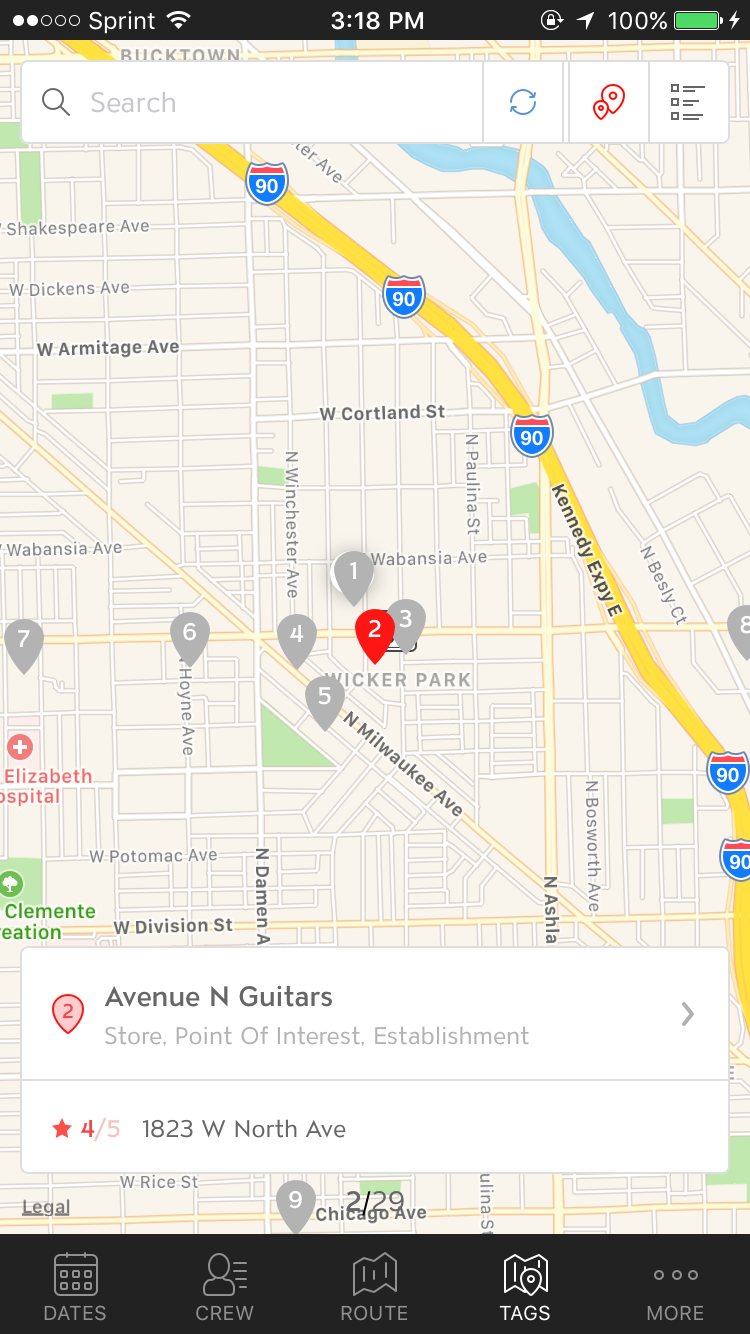The image is a detailed screenshot taken from a smartphone. In the top left corner, there are two solid circles and three hollow ones, likely representing signal strength. The time displayed is 3:18 PM, and the battery indicator shows a full charge at 100%. A green search bar is present with a refreshed command. Below, there is a map featuring multiple pins and various points of interest.

The map showcases the 90 Freeway, also known as the Kennedy Expressway, running east-west. Nearby streets include Clifton Street and West Armitage Avenue. There are seven pins on the map, indicating locations of interest. In the bottom left corner, notable places marked include Elizabeth Hospital, Clements Station, and West Division Square.

At the bottom of the map, a red pin marks a specific location near Texas Avenue and a guitar store, noted as a point of interest or establishment. The map also highlights a highly rated area with a review of four to five stars at 1823 West North Avenue.

Additional elements on the screen include tabs displaying "dates," "calendars," "crew," "Drew," and "tags," with Dawson mentioned as well. Lastly, a river is visible in the top right corner of the map, intersecting various streets and roads.